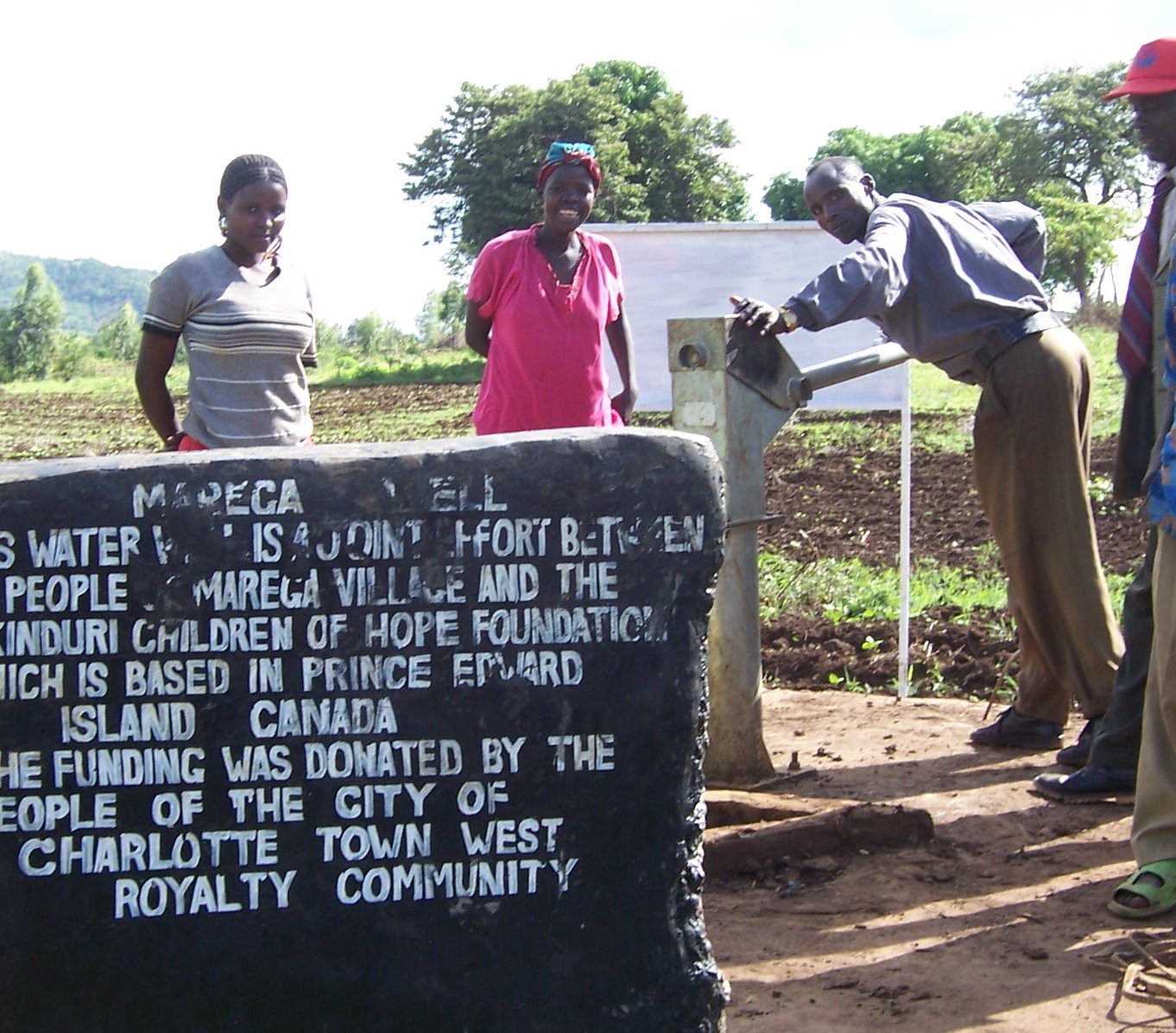The photograph depicts a group of four people standing by a public water pump, likely part of a recent fundraiser in an African village. Central to the image is a man actively pumping water from a metal device. Two women, one in a gray shirt and one in a pink shirt, both with short hair, stand on the left side, while two men are on the right, one in a work dress shirt and brown pants, the other wearing a pink hat and a tie. The background features a field with dark earth, scattered plants, and large trees under a vast sky. In the foreground, a large, flat, dark stone bears text slightly obscured by age, indicating a joint effort between the people of Moraga Village and the Kinduri Children of Hope Foundation, supported by donations from the community of Charlottetown West Royalty, Prince Edward Island, Canada. The scene is set in the daytime, highlighting the rural and communal atmosphere.